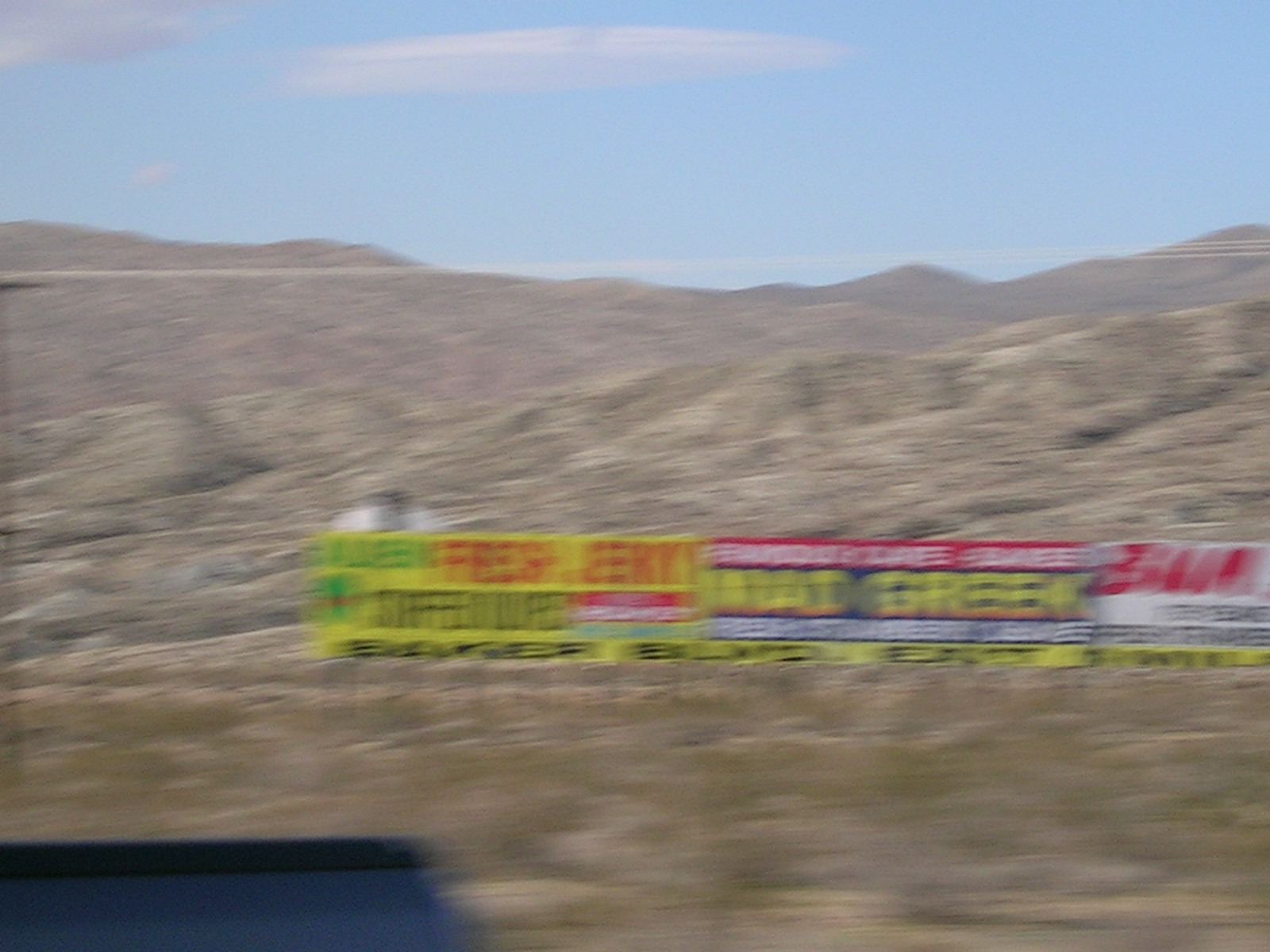Captured from a rapidly moving vehicle, this photograph encapsulates the essence of the Southwestern United States, reminiscent of the storied Highway Route 66 traversing through Arizona, New Mexico, or approaching California. The motion blur of the image results in a dreamlike quality, rendering long road signs and distant billboards nearly unreadable. However, certain signs are legible, including one advertising "beef jerky" and another marked "creek." The remaining signs fade into a haze of speed-induced blur.

In the background, the landscape unfolds into dry, arid terrain characterized by mountainous and eroded hillsides. Sagebrush patches sporadically dot the scene, contributing to the unmistakable Southwest ambiance. A smooth-topped mountain stands tall against the clear blue sky, punctuated by a smattering of clouds. The overall vista captures a timeless moment on the fabled highway, invoking the classic feel of an endless road journey through America's rugged desert heartlands.